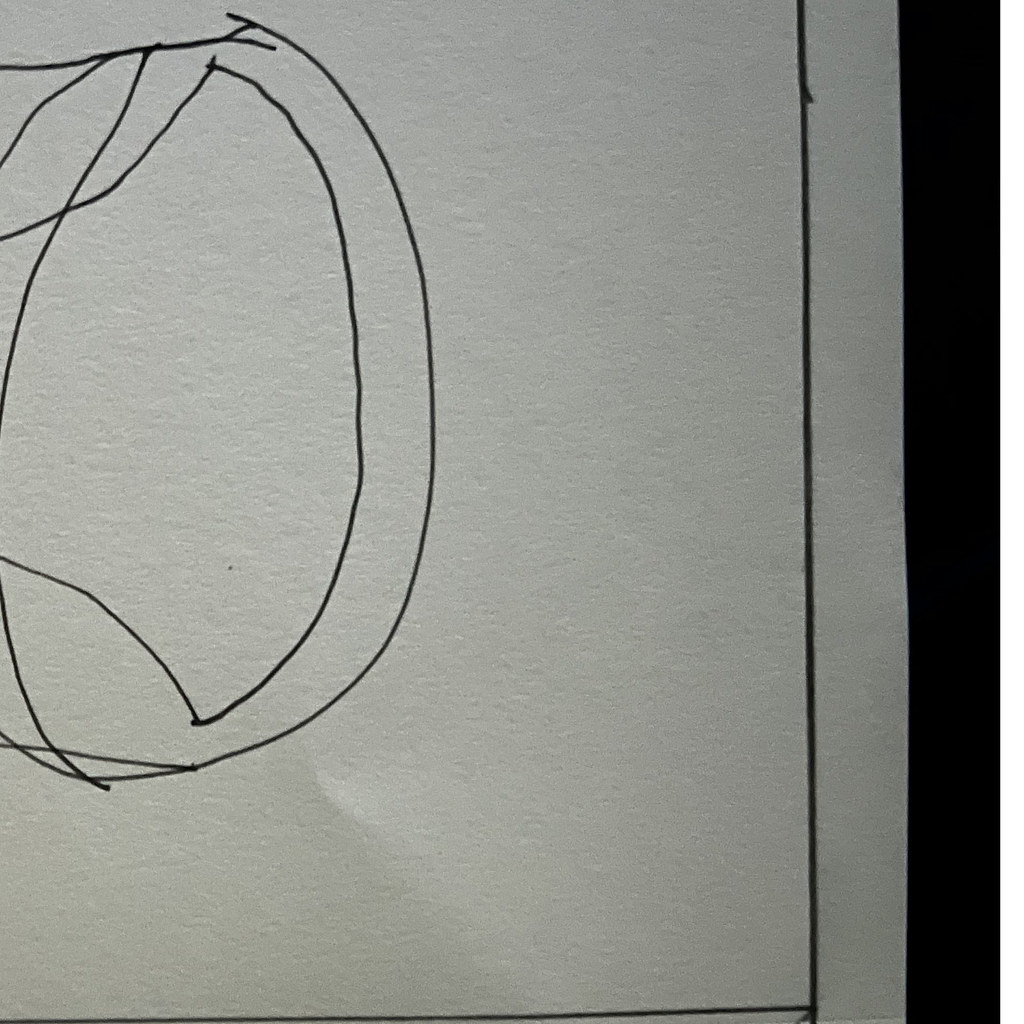The image features a complex design with multiple geometric elements and intricate lines. On the right-hand side of the image, there is a vertical black rectangle. Adjacent to the rectangle is a gray area that transitions into another horizontal black line. This horizontal black line intersects with a perpendicular black line, forming a cross-like structure. The background appears to be a whitish gray, resembling paper.

Within this structured layout, a squiggly drawing captures attention. At the top of this drawing, there is a line that descends and then forms an inverted or sideways "V" on the left-hand side. The line then continues, creating a "Z" shape before curving all the way around to the left-hand side of the paper. There's another line within this squiggly drawing that stretches from the left edge to the outer rim of the structure. 

Additionally, a separate line begins at the top of the drawing and goes off-screen to the left, reappearing further down. This line extends slightly past the previously mentioned curve. A distinct bell-shaped line begins at the left-hand side, curving upward and outward before forming a roundish curve and finally inclining inward where it exits the paper on the left-hand side.